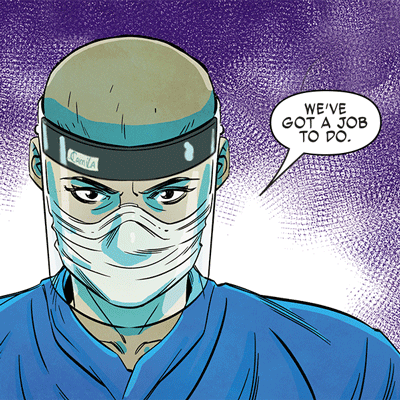The image is a cartoon style illustration with a textured, purplish background, as if created by rubbing a purple crayon over burlap. It features a serious-looking healthcare worker adorned in blue scrubs, a face shield, and a face mask highlighted in blue. The worker, potentially a heroic figure, has a square jawline visible beneath the mask and light brown hair that might be partially covered by a surgical cap. Piercing eyes and furrowed brows add to their determined expression. A white speech bubble to the right, pointing towards the worker, contains the text "We've got a job to do" in black lettering. The panel suggests a pandemic-era setting, emphasizing the worker's readiness for a critical task, likely in a medical or surgical context.